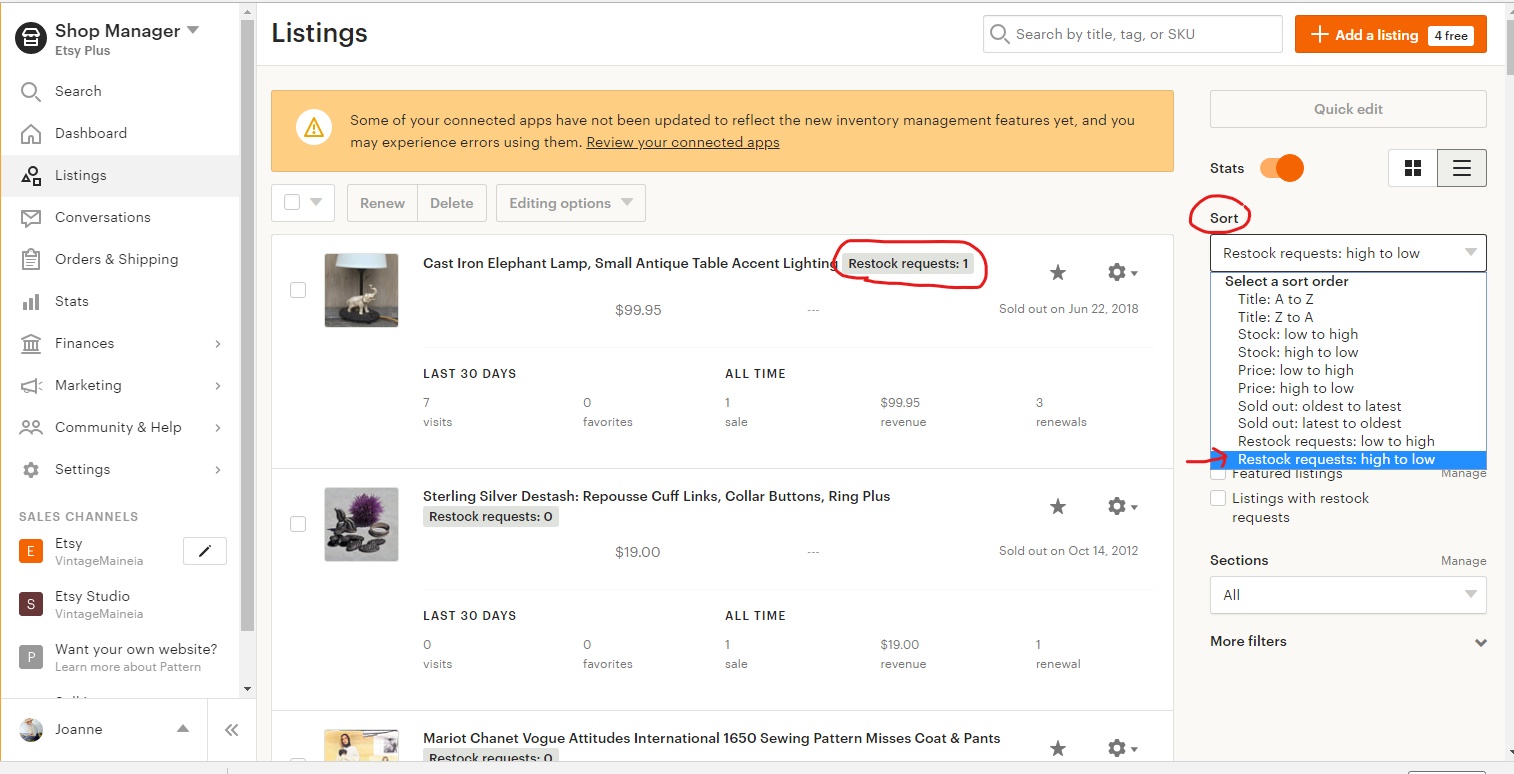This detailed caption describes a screenshot of a seller's dashboard on Etsy's website:

---

This color photograph captures a screenshot of an Etsy seller's dashboard. The webpage has a predominantly white background, and the upper left-hand corner features the headline "Shop Manager," followed by the "Etsy Plus" logo. The left sidebar presents a list of navigational items, including Search, Dashboard, Listings, Conversations, Orders and Shipping, Stats, Finances, Marketing, Community and Health, and Settings.

The central portion of the page, which occupies about three-quarters of the layout, is dominated by the "Listings" section. At the very top left of this section is a light orange rectangle containing a warning message. This rectangle includes a white circle with a black exclamation point inside, indicating a warning. The message reads: "Some of your connected apps have not been updated to reflect the new inventory management features yet, and you may experience errors using them." Below this, an underlined text prompts the user to "Review Your Connected Apps."

Further down in the listing section, two items are prominently displayed, with part of a third entry visible. The first listing is titled "Cast Iron Elephant Lamp," accompanied by a small image depicting a lamp with an elephant figure at its base. The second listing, "Sterling Silver D-Stash," showcases an image of cufflinks.